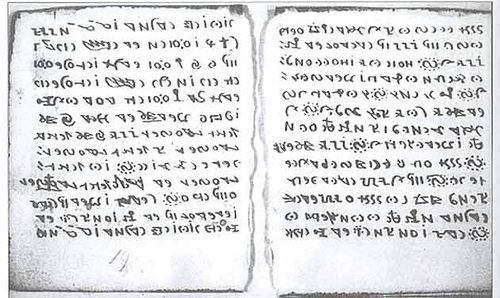The image depicts two torn photocopies of documents split down the middle, each covered in lines of random symbols with no discernible punctuation or readable language. The photocopies exhibit characteristic ink shading around the edges, highlighting their reproduced nature. The margin distribution suggests the papers are oriented upside down, with a narrow margin visible at the top edge and a larger margin at the bottom. The nonsensical nature of the writing implies these pages contain fabricated text rather than any meaningful content.